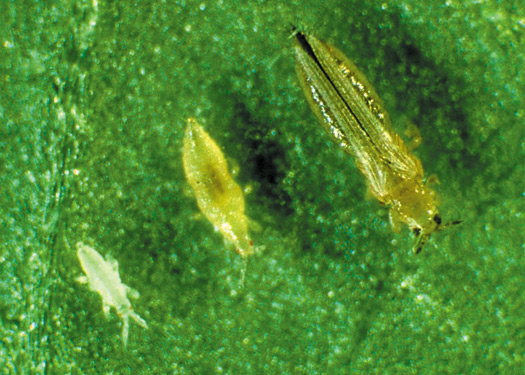The close-up photograph captures three different stages of an insect's life on a vibrant green, spotted leaf. From left to right, the insects increase in size and maturity. The smallest, nearly translucent insect on the bottom left has faint, light features and tiny antennas. The middle insect is slightly larger, yellowish-green, and semi-transparent with noticeable reddish eyes. The largest insect on the far right is fully developed, predominantly yellow-green with pronounced black eyes and a distinct black stripe running down its back. Each insect is shown in impressive detail, highlighting the progression of its growth stages.